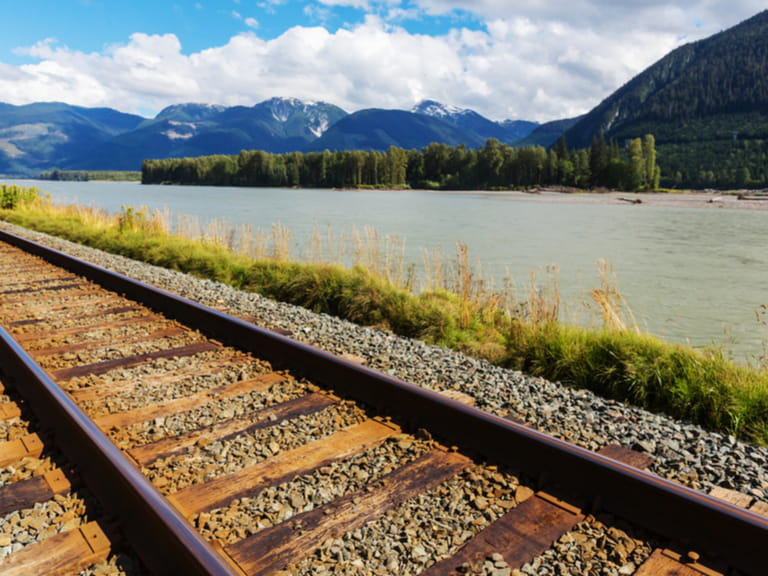This detailed, photorealistic landscape photograph features weathered, rusted railway tracks running from the lower right foreground, diagonally upwards and left, gracefully diminishing in perspective. The tracks, perched on old wooden crossbeams over a rocky gravel bed, lay mere feet from the edge of a large, serene body of water. A thin line of grasses and some shrubbery form a natural border between the gravel and the water. The calm water surface, adorned with slight ripples, stretches smoothly toward a dense stand of pine trees on the far shore. Above the trees rise majestic blue mountain ranges, with a few snow-capped peaks hinting at their elevation. The vivid, bright blue sky is dotted with fluffy, thick white clouds, adding depth to this tranquil, undisturbed scene. The photograph captures a serene moment, devoid of any visible animal life or human presence.